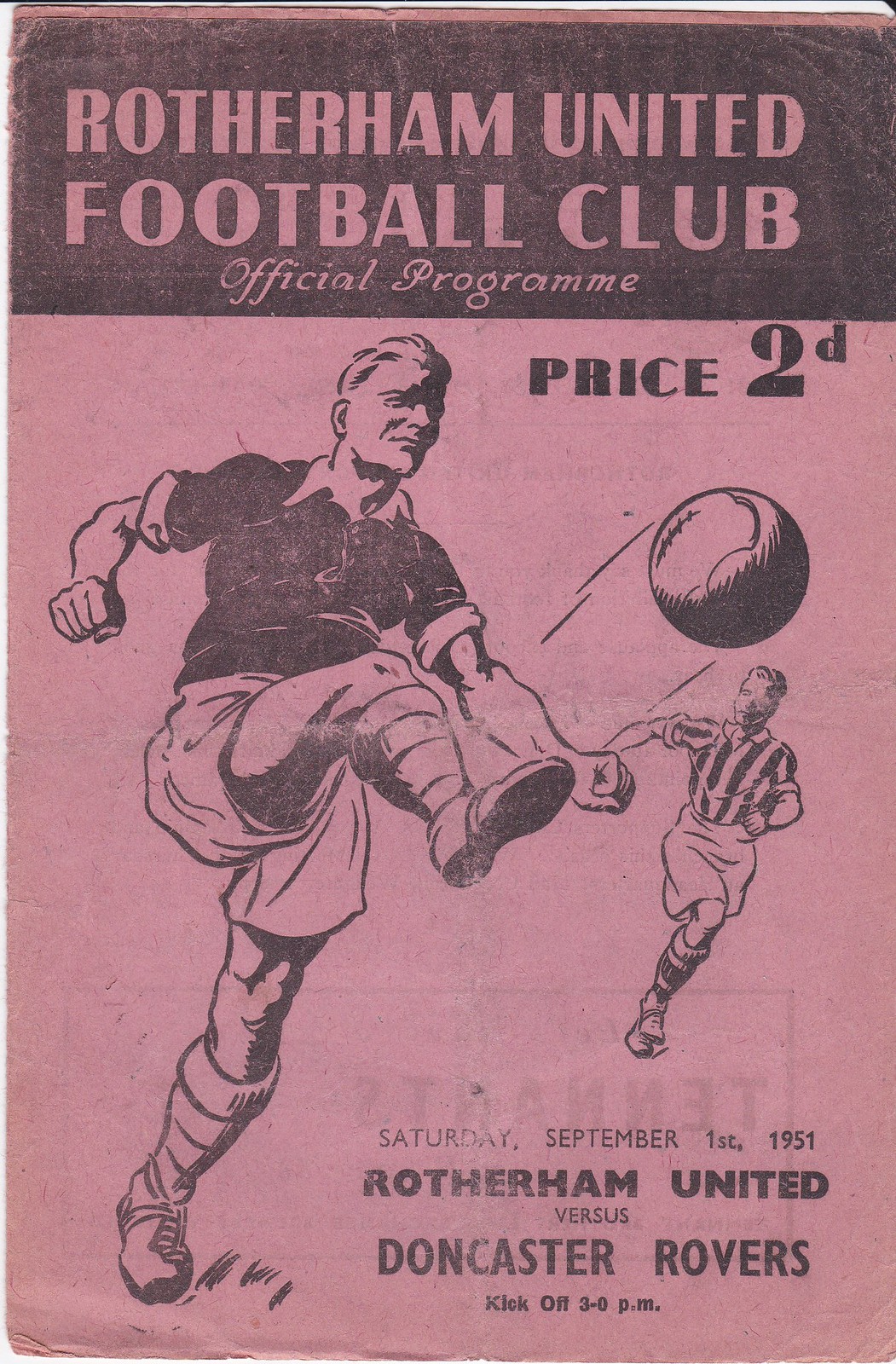This cover of an official program from Rotherham United Football Club, dating back to September 1st, 1951, features a worn, dark pink background indicative of its aged condition. The top 25% of the cover showcases a horizontal black bar with pink text that reads "Rotherham United Football Club Official Program." On the upper right corner, in black text against the pink background, it states "Price 2D." A black and white sketch dominates the lower portion of the cover, depicting a footballer mid-action, kicking a soccer ball. The player is dressed in a black shirt, white shorts, white socks, and cleats, with a referee in a striped shirt and white shorts trailing behind. Below this illustration, in the lower right corner, the details of the match are clearly displayed: "Saturday, September 1st, 1951, Rotherham United versus Doncaster Rovers, kickoff 3 p.m." The overall condition of the program shows its age, with visible faded print, worn lines, and creases that suggest it has been folded and well-handled over the years.